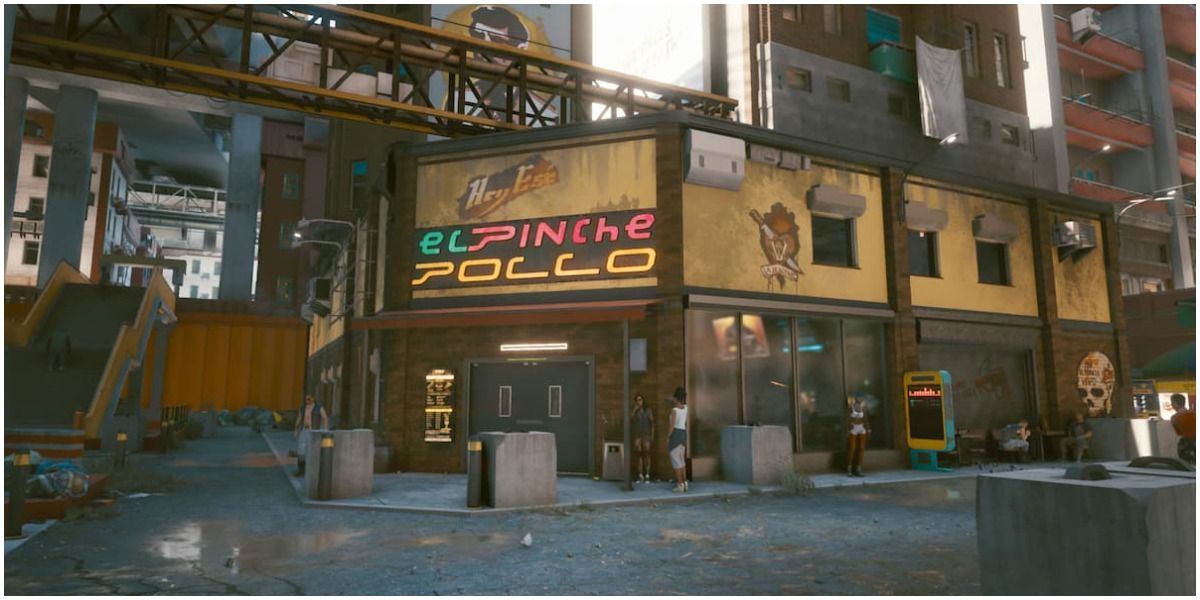The image depicts a corner building that appears to be from a video game or animated scene. The structure itself is a two-story establishment called "El Pinche Pollo." Its signage is prominently lit, with "El" in blue, "pinche" in pink, and "pollo" in yellow lighting. The building's facade features a tan upper portion and a brown lower section, punctuated by numerous windows. A door on the right has a light above it, with a skull drawing visible on the building's far right side. The left side reveals a staircase leading to another area, seemingly to a higher street level. A few people are seen mingling around the entrance, and some outdoor tables and chairs suggest it functions as a restaurant. The background shows a high-rise apartment building with visible balconies, adding an urban context. The street and immediate surroundings appear dilapidated, with cracked pavement and scattered trash, contributing to a dark, seedy atmosphere.